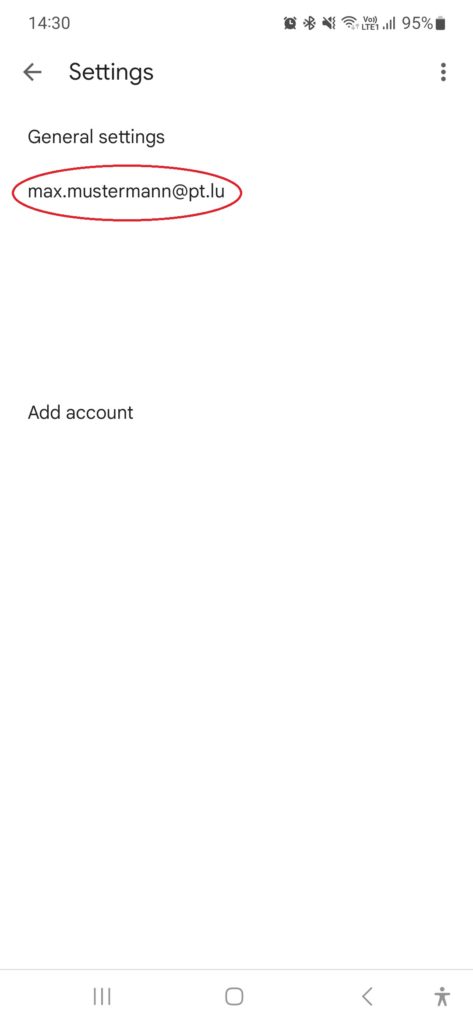This image is a screenshot captured from someone's phone, showcasing specific user interface elements. In the upper left-hand corner, the time is displayed as 14:30. On the upper right-hand corner, multiple status icons are present, with the last one being a battery icon indicating a 95% charge. Beneath this icon, there is a vertical row of three small dots.

Directly under the time, a left-pointing arrow and the word "SETTINGS" are prominently displayed. Below "SETTINGS," the smaller-font text "GENERAL SETTINGS" is visible. Further down, an email address, "MAX.MUSTERMANN at PT.LU," is prominently featured and circled in a red oval, emphasizing its importance.

Centered in the middle of the screenshot, the option "ADD ACCOUNT" is clearly displayed, suggesting an interactive element for adding new accounts. 

At the very bottom of the image, a thin gray line separates the central content from the navigation bar, which contains four icons: a menu represented by three lines, an application grid symbolized by a square, a back arrow pointing left, and a user profile icon depicting a person. The background of the screenshot is white, with all text rendered in black or gray tones, ensuring clear visibility and readability.